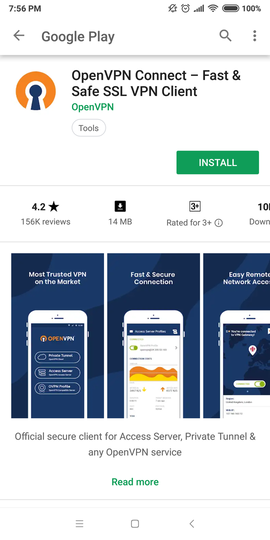In this image, the Google Play Store interface is displayed, showcasing the "OpenVPN Connect – Fast and Safe SSL VPN Client" application that is in the process of being installed. At the very top, "Google Play" is prominently displayed. Below that, on the top left, the application's name "OpenVPN Connect – Fast and Safe SSL VPN Client" is written in black text. Directly underneath, in green text, is "OpenVPN," with the category "Tools" labeled beneath it.

To the left of this text, there is an app icon featuring an orange outer ring and a blue keyhole set against a white background. 

On the right side in the center, there is a prominent green "Install" button with "Install" written in white. Below this button is a brief description of the app which highlights its 4.2-star rating based on 156,000 reviews. The app's size is 14MB, and it is rated as suitable for ages 3 and up.

Further down, the image shows three screenshots of the app displayed within a smartphone frame. These screenshots have a blue background. The first screenshot, positioned on the left, claims "Most Trusted VPN on the Market." The second screenshot, located centrally at the bottom, states "Fast and Secure Connection." The third screenshot to the right says, "Easily Remote Network Account."

Towards the bottom of the image, it reads "Official Secure Client for Access Server, Private Tunnels and any OpenVPN Service." Finally, a green "Read More" button appears at the very bottom, inviting users to learn more about the application.